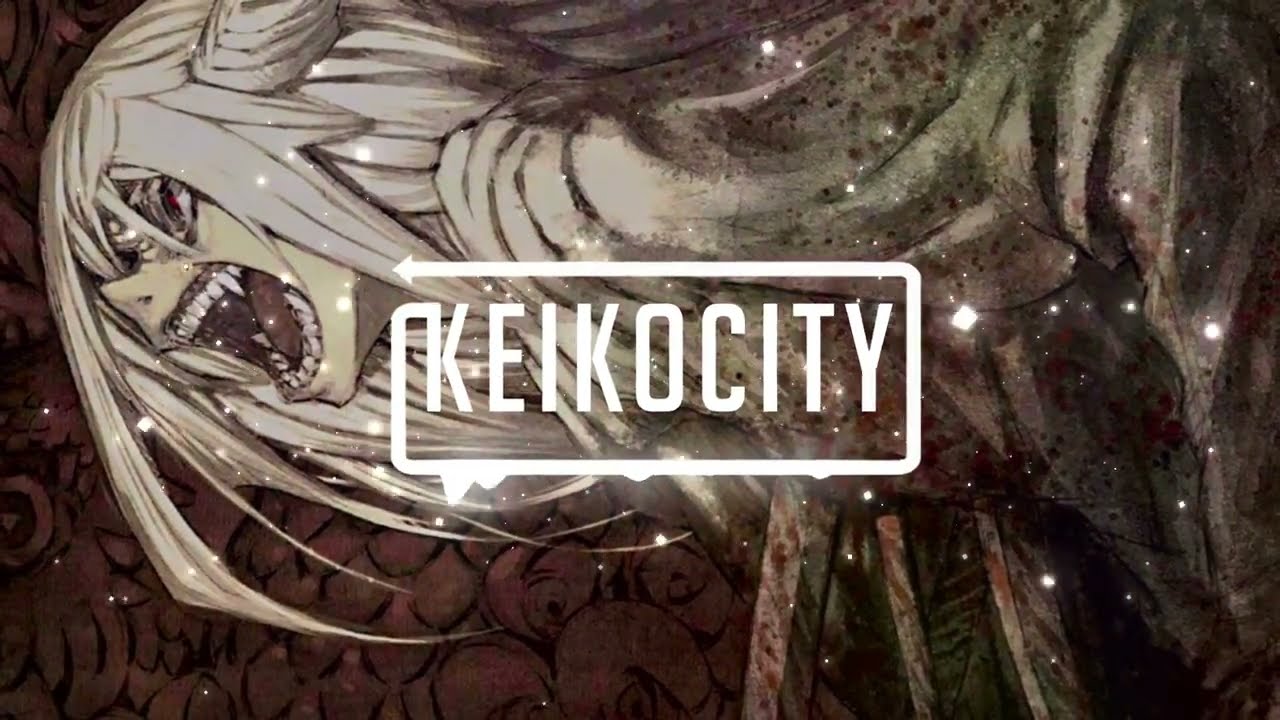The horizontally rectangular digital image prominently features a logo in the center with the text "KEIKOCITY" in bold block letters. Encircling the text is a unique frame forming a box: the top section extends into a leftward-pointing arrow. In the main visual, there's a vividly drawn Anime character, depicted at a 45-degree angle with a dramatic, expressive pose. This character has an elongated head projecting leftward, revealing a wide, menacing mouth filled with sharp vampire-like fangs and square teeth between them. The mouth is open in an intense, angry growl. Covering the character's face partially are strands of jagged, long white hair that cascade down their sides and across their forehead, partially obscuring fierce red eyes. The character's light-colored skin contrasts sharply with the blood-spattered white cloak they are wearing. The background of the image is textured with scales, reminiscent of fish or dragon scales, adding to the dynamic and fantastical theme of the artwork.